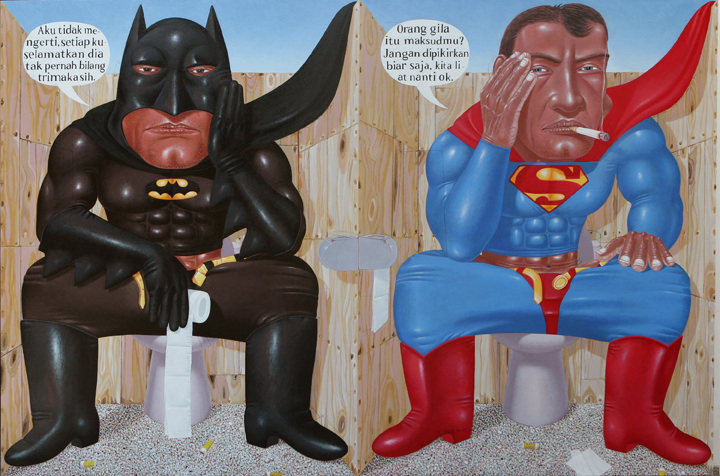In the image, Batman and Superman are depicted in a unique, cartoonish art style, sitting on toilets within wooden bathroom stalls. Batman, positioned on the left, has his left elbow resting on his knee and his hand cupping his cheek, exuding a contemplative demeanor. He holds a roll of toilet paper, seemingly taken from the dispensers in the stall. A word bubble in a foreign language with grey writing hovers next to him. Batman is dressed in his traditional black suit, mask, cape, and thick boots, his muscular build clearly outlined.

Superman, seated on the right, mirrors Batman's pose, with his right elbow on his knee and his cheek resting on his hand. A lit cigarette dangles from his mouth, reinforcing a more rugged appearance. Another word bubble, also in a different language and grey writing, is near him. Clad in his iconic blue and red suit, his belt is undone. The bathroom floor is cluttered with rolls of toilet paper and cigarette butts, adding to the chaotic scene. Above the stalls, a clear blue sky is visible, contrasting with the otherwise confined setting.